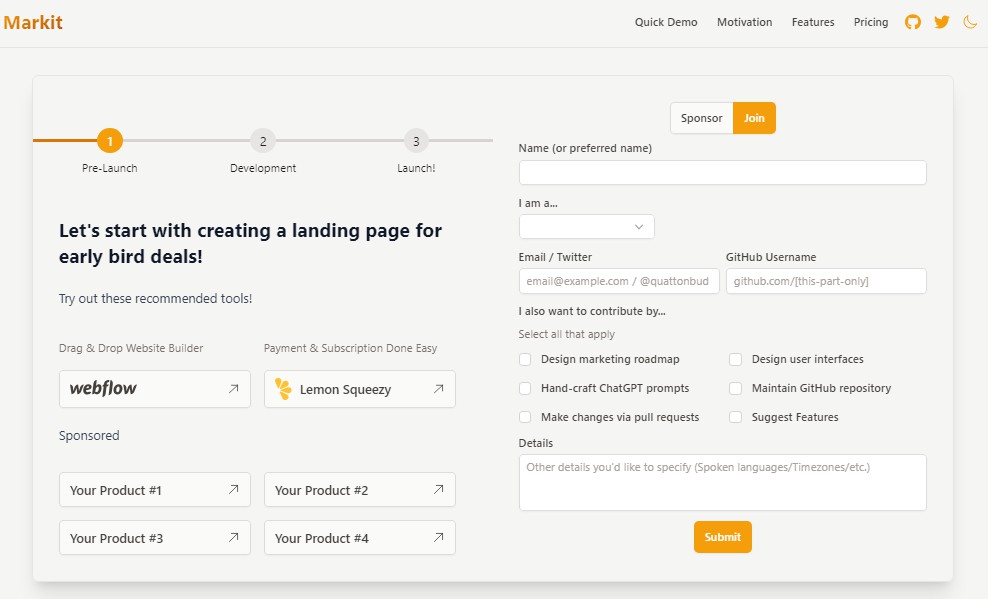Sure, here is a more detailed and cleaned-up version of the caption:

---

The image features a structured landing page with a gray background and several outlined sections in orange. At the top, the header includes categories titled "Market," "Quick Demo," "Motivation," "Features," and "Pricing." On the left side, there are familiar icons: a Reddit symbol, a Twitter logo, and a moon. 

Beneath these icons, a section is depicted as a lawn with three distinct phases marked by numbered labels: an orange "1" for Prelaunch, a gray "2" for Development, and another gray "3" for Launch. Each phase has its own detailed explanation below it, likely outlining the steps involved.

In the center of the page, a white rectangle with the word "Sponsor" in black is prominently displayed, followed by an orange rectangle also labelled "Sponsor." Further down, there is another orange rectangle containing the word "Join" in white text.

Below this, there is a registration box requesting information such as "Name (or Preferred Name)" marked with "IMA," "Email/Twitter," "GitHub Username," and a checkbox section labeled "I also want to contribute by." The options available to select include: Design, Marketing Roadmap, Handcrafting ChatGPT Prompts (in all capital letters), Making Changes via Pull Requests, Designing User Interfaces, Maintaining the GitHub Repository, Suggesting Features, and a details section with an input box.

The bottom of the page features a large orange rectangle with the word "Submit" in white, indicating a call to action. The caption suggests that the page is intended to introduce early bird deals and recommended tools, with additional explanations provided for users to understand the benefits and steps involved.

---

This formulation should provide a clear and comprehensive picture of the webpage layout and its key elements.